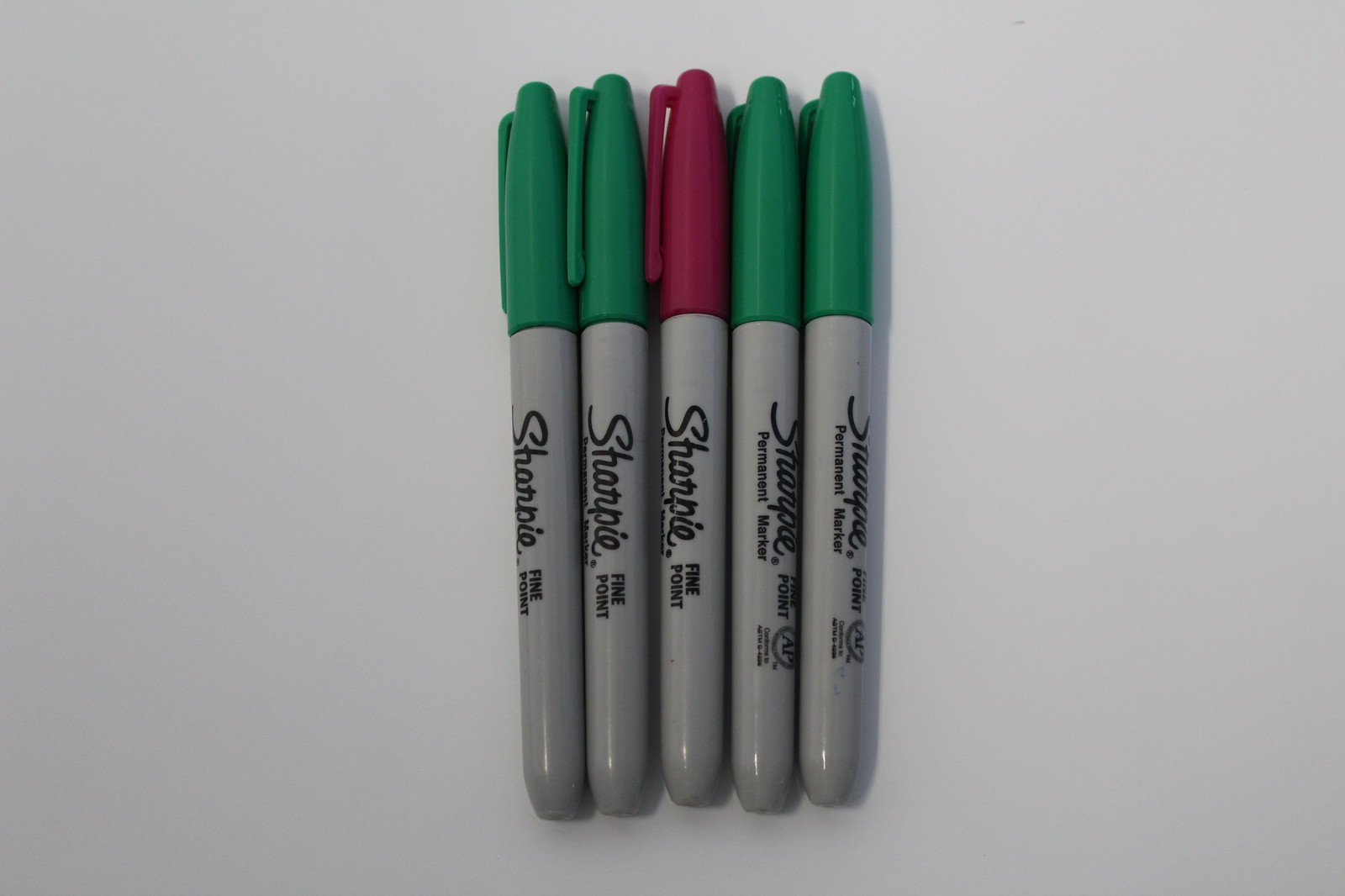The image captures a row of five Sharpie markers on a flat white countertop. Four of the markers have green caps, while one stands out with a red cap positioned centrally. The arrangement is symmetrical, with two green-capped markers on either side of the red-capped one. Each marker features a gray barrel with the word "Sharpie" inscribed in black script, along with the words "Fine Point" nearby. Among these, two markers display a trademark logo adjacent to the "Fine Point" label, while three do not. The markers are aligned in a fairly straight line, with slight variations in positioning. The overall composition creates a balanced and visually striking contrast reminiscent of festive, Christmas colors.